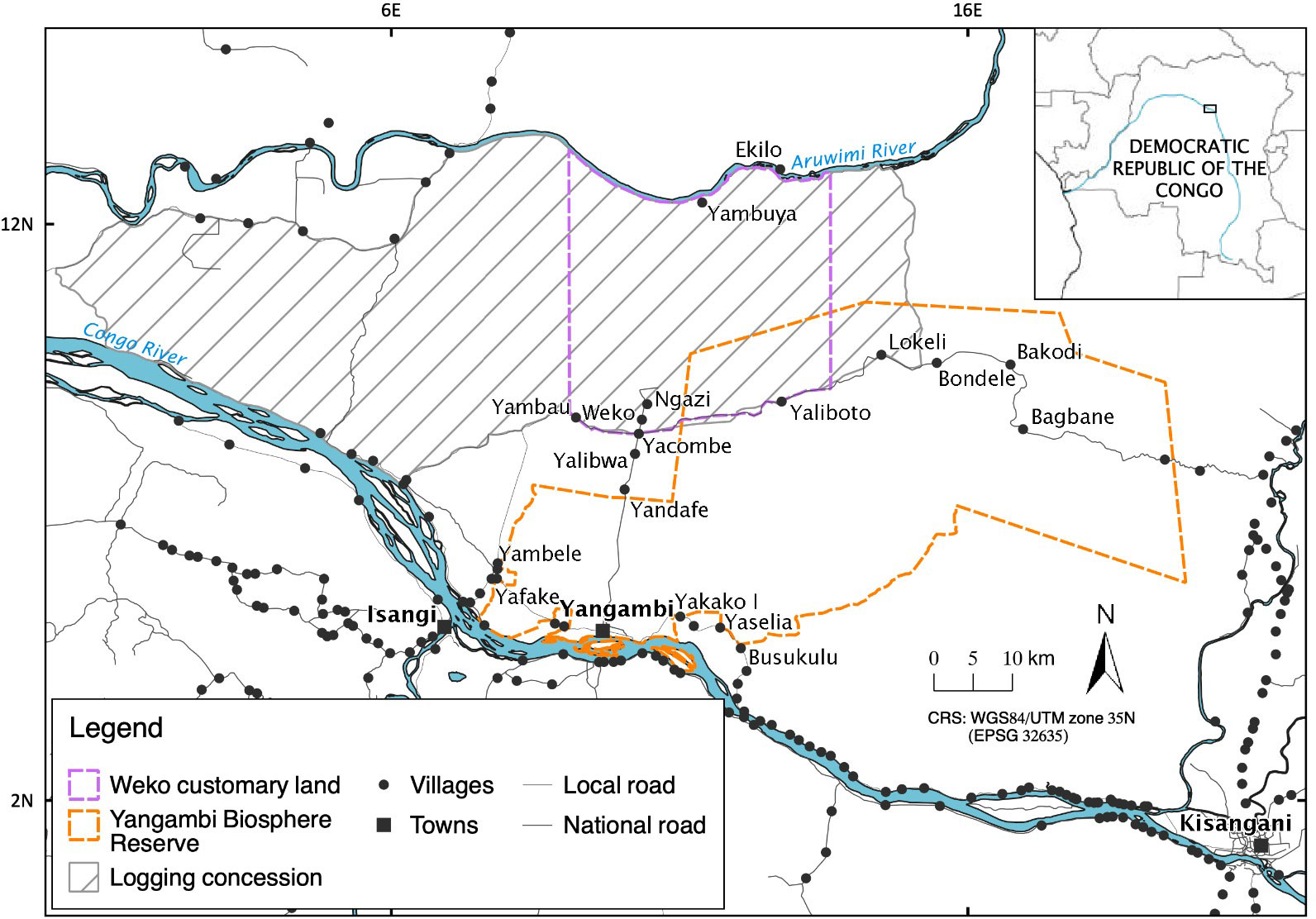A detailed map of the Democratic Republic of the Congo is displayed on a white background. In the top right corner, a squared-off section marks the country's name. The map showcases numerous blue rivers, with a prominent one surrounded by black dots representing various towns and villages. Local and national roads are highlighted in brown. Weko Customary Land and the Yangambi Biosphere Reserve are marked alongside logging concessions. Purple diagonal stripes with dotted lines and an orange dotted shape signify specific regions or boundaries. Cities and villages are labeled in black text, with larger font for significant towns such as Yambeli, Yandafi, Yacombi, Ngozi, Yaloboto, Locale, Blondel, and Bakodi. In the bottom left corner, a legend within its own rectangle explains the map's various symbols and scales, providing a comprehensive reference for distance and regional delineations.